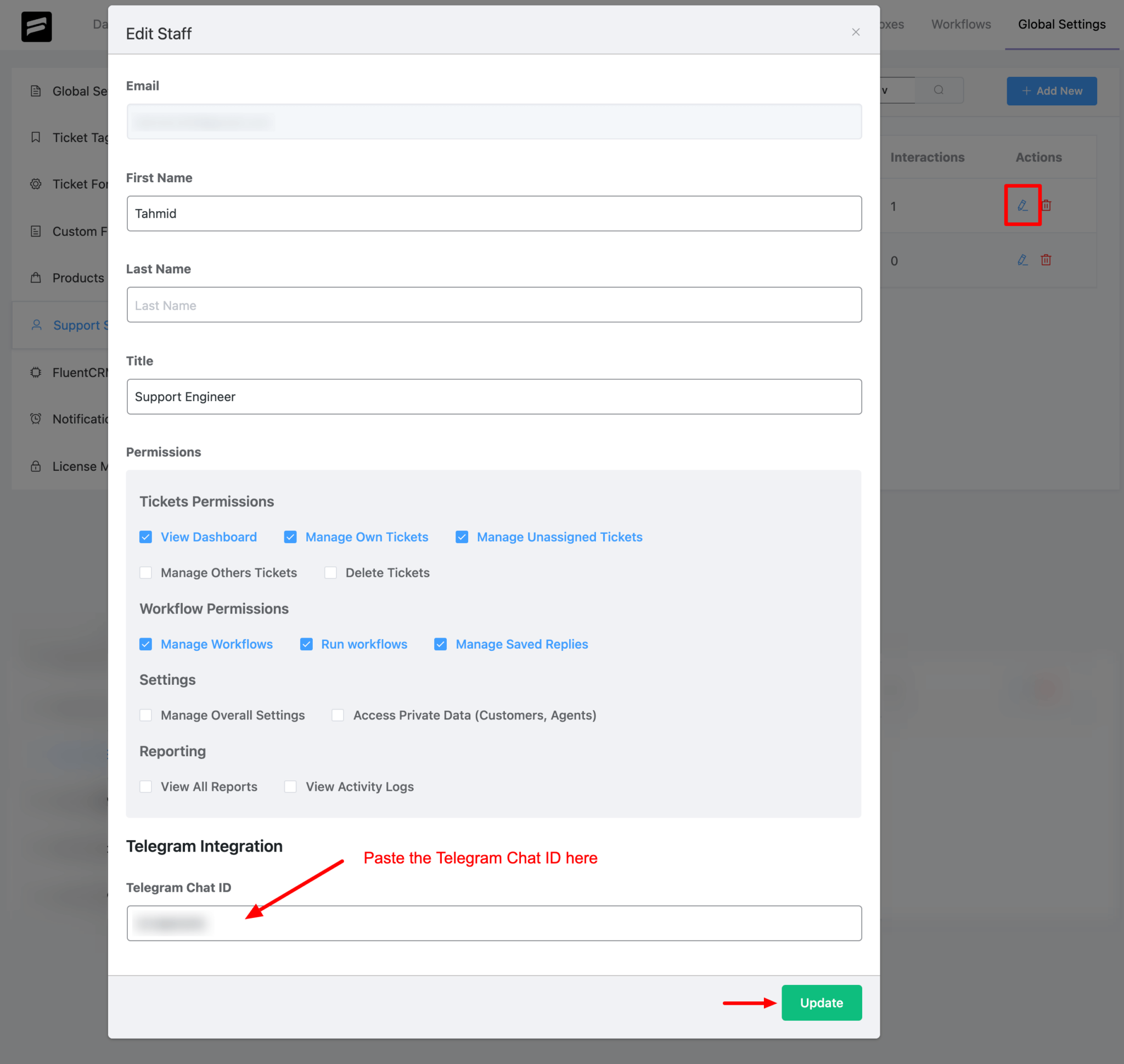This image captures a screenshot of a web page subpage, likely part of a complex web application, rather than an iPhone interface. The main webpage serves as a dashboard for managing various settings and workflows, and the subpage is designed for editing staff details and permissions.

In the subpage, the top left corner features a black and white logo, with the entire subpage overlaid by a subtle gray filter. On the right side, partial text indicates sections labeled "Workflows" and "Global Settings," though the rest is not visible. Directly below these sections is a prominent blue button labeled "Add New." Underneath the button are two columns: one titled "Interaction" and the other "Actions." The "Interaction" column lists "One Interaction" followed by several icons representing actions, while the "Actions" column shows "Zero Interaction" and subsequent symbols.

On the left side of the main webpage, there are truncated navigation options, listing items such as “Global,” partially shown as "SE," "Ticket TA," "Ticket FO," "Custom F," "Products," "Support," "Fluent CR," "Notifications," and "License."

Within the main content of the subpage, a window titled "Edit Staff" is visible, featuring a top-right hand 'X' for closing the window. This window asks users to "Fill in the boxes." The fields include "Email," a "First Name" field already filled in as "Tomid," a blank "Last Name" field, and a titled "Support Engineer" with various permission settings. 

Permissions are categorized into three sections:
1. **Ticket Permissions**:
   - Checked: View Dashboard, Manage Own Tickets, Manage Unassigned Tickets
   - Unchecked: Manage Other Tickets, Delete Tickets

2. **Workflow Permissions**:
   - Checked: Manage Workflows, Run Workflows, Manage Saved Replies

3. **Settings**:
   - All unchecked: Manage Overall Settings, Access Private Data, Customer Agents, Reporting, View All Reports, View Activity Logs

Below these permissions, there is an area for "Telegram Integration," featuring a Telegram chat ID input box, which is currently blurred out. A red arrow directs the user to paste the Telegram chat ID into this box, with another red arrow pointing to a green "Update" button located in the bottom right corner, indicating the final step to save the changes.

This detailed screenshot provides a comprehensive view of the workflow management and permissions set within the application, enhancing user control and customization in the support staff editing process.